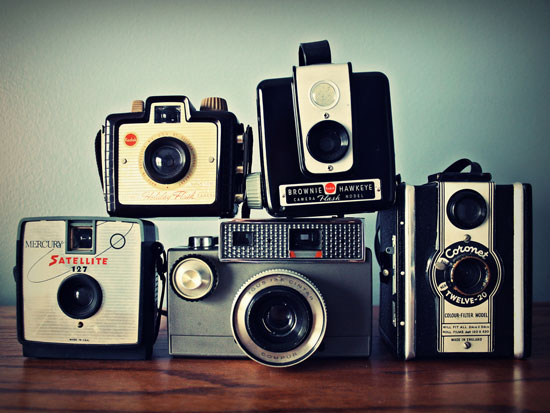This image, likely a slide from the 1950s or 1960s, showcases a collection of five vintage cameras arranged in a stacked formation. The setting is a wooden table of muted brown, with a plain white background. The overall photograph has a cyan tint, suggesting age. The cameras include prominently displayed Brownie models, with specific branding visible such as "Mercury Satellite" and "Brownie Hawkeye." The arrangement features three cameras on the bottom and two boxy Brownie cameras stacked on top. Each camera, primarily in black, white, and silver, is oriented to face the viewer, highlighting their old-fashioned designs. This photo, possibly taken as a catalog or sales image, captures the nostalgic essence of these well-preserved, mid-century manual film cameras.